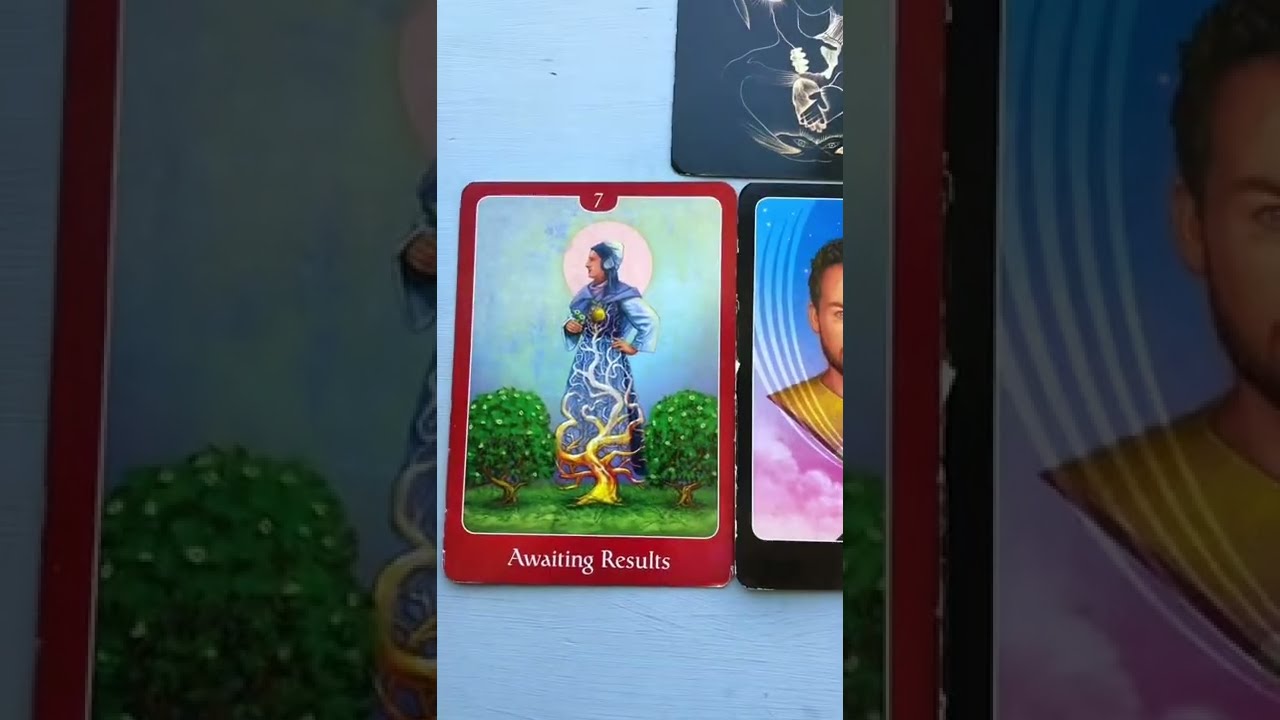The image is a wide rectangular collage featuring a tall rectangular photograph of cards at its center, flanked by darker, slightly wider cropped sections of the same photograph on both sides. The background of the photograph is a light blue surface. The central focus is a fully visible card with a red border, depicting a woman in a multicolored blue outfit. She is connected to a yellow-white tree, with her body entwined by its branches and roots. She stands in front of a glowing pink moon, and there are two small green bushes beside her. The card has the text "Awaiting Results" at the bottom and a white number seven at the top.

On the right side of the central card, a portion of another card is visible, featuring a man with a pink cloud beneath him, set against a purple and light blue sky. Additionally, there is a partially visible black card at the upper right, showing hands holding other hands. The image overall creates a mystical scene with interconnected elements and a serene, contemplative atmosphere.